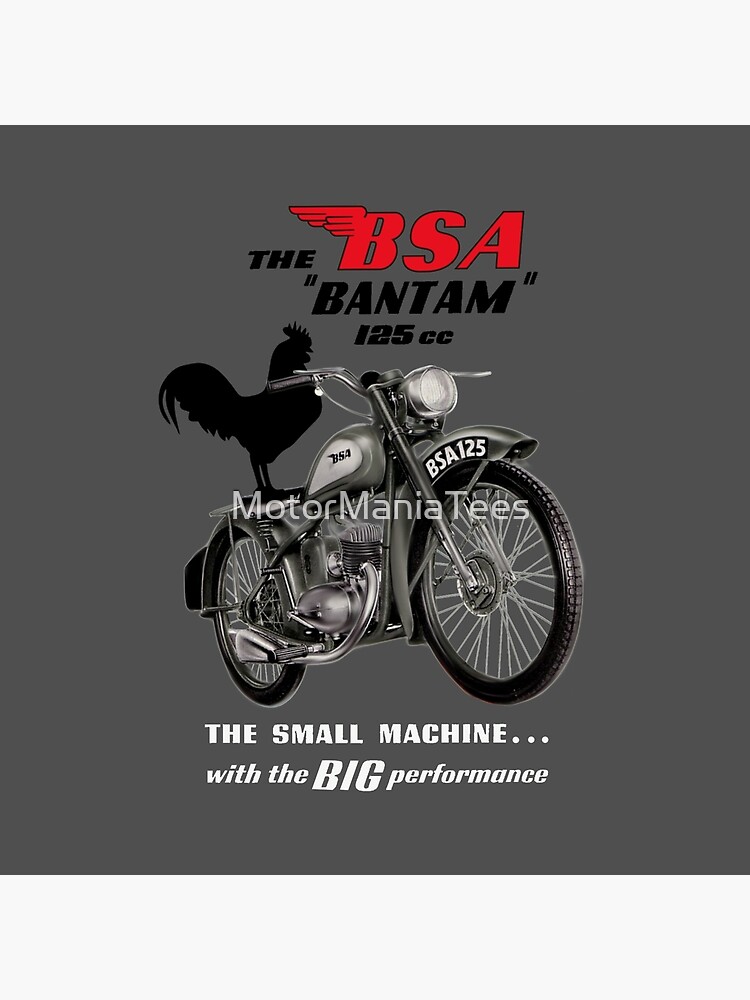This rectangular advertisement, measuring approximately 5 inches high and 4 inches wide, features a light gray header and footer, each about 3/4 of an inch in height. The main body of the image has a dark gray background, with an old-fashioned motorcycle prominently displayed in shades of gray at the center. The motorcycle is detailed with shiny silver spokes, tires, a large headlight, and both front and rear fenders. 

At the top center of the image, bold red letters outlined in black spell out "BSA", with an angel's wing extending from the upper left corner of the "B". Just below this, in black print, it reads, "The Bantam" followed by "125cc". A black silhouette of a rooster perches on the back seat of the motorcycle, adding a unique touch. 

Across the front of the motorcycle, the text "Motor Mania T's" is written in light blue. Beneath the motorcycle, the slogan "Small engine with the big performance" underscores its capabilities. Overall, the advertisement combines nostalgic style with modern touches, emphasizing the motorcycle's compact yet powerful engine design.